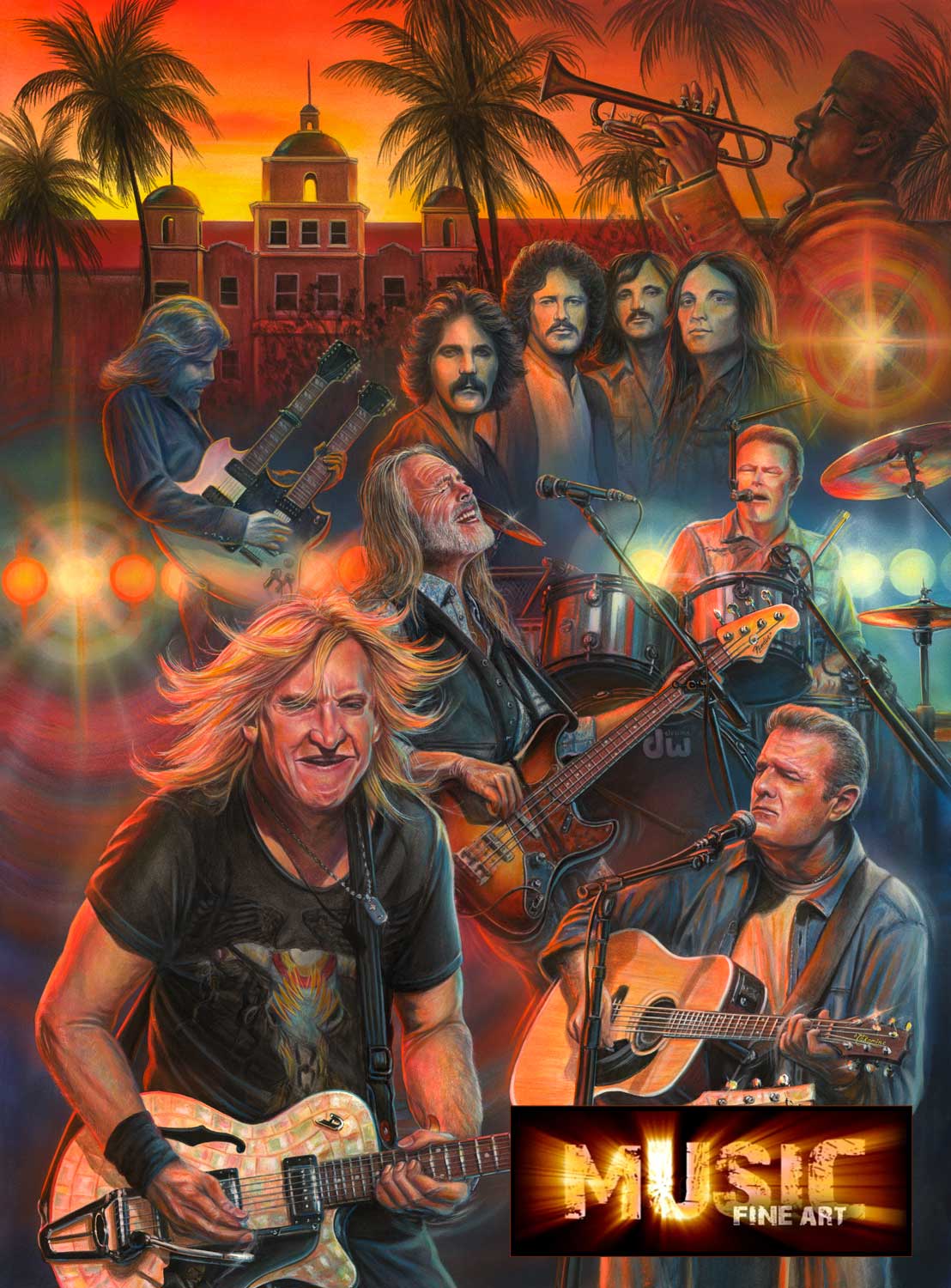This hand-illustrated music poster vividly captures a dynamic group of musicians amid a vibrant outdoor and indoor setting, blending elements of both scenes harmoniously. The background features a warm, orange-yellow sunset sky, accentuated by a couple of palm trees and a prominent domed building, lending an atmospheric depth to the image.

In the top right corner, the legendary Louis Armstrong is depicted in near black-and-white tones, playing his trumpet to the left. Just below him, a quartet of young musicians with long black hair and mustaches stand solemnly, their static presence contrasting with the energetic figures around them.

At the forefront, a striking white man, possibly in his 50s, stands out with his long flowing blonde hair and a black graphic shirt, deeply engrossed in playing an electric guitar adorned with a mosaic pattern. Beside him, a man with short slicked-back hair, wearing a black jacket, focuses intently on his acoustic guitar, his mouth poised near a microphone ready to sing.

In the middle section, a gray-haired, bearded man passionately plays an electric guitar, his head tilted upward, eyes closed in musical reverie. To his right, a drummer in a brown shirt simultaneously plays and sings into a microphone attached to a headset, adding an additional layer of complexity to the composition. Behind these central figures, a double-necked guitar player with dark wavy hair leans back, fully immersed in his performance.

Adding to the layered character of this scene, a man sitting on the ground to the left, with blonde hair and a gray jacket, strums his acoustic guitar, contributing to the overall musical synergy.

In the bottom right corner, the text "Music Fine Art" discreetly anchors the piece, reinforcing the artistic and celebratory essence of this richly detailed, illustrative poster.